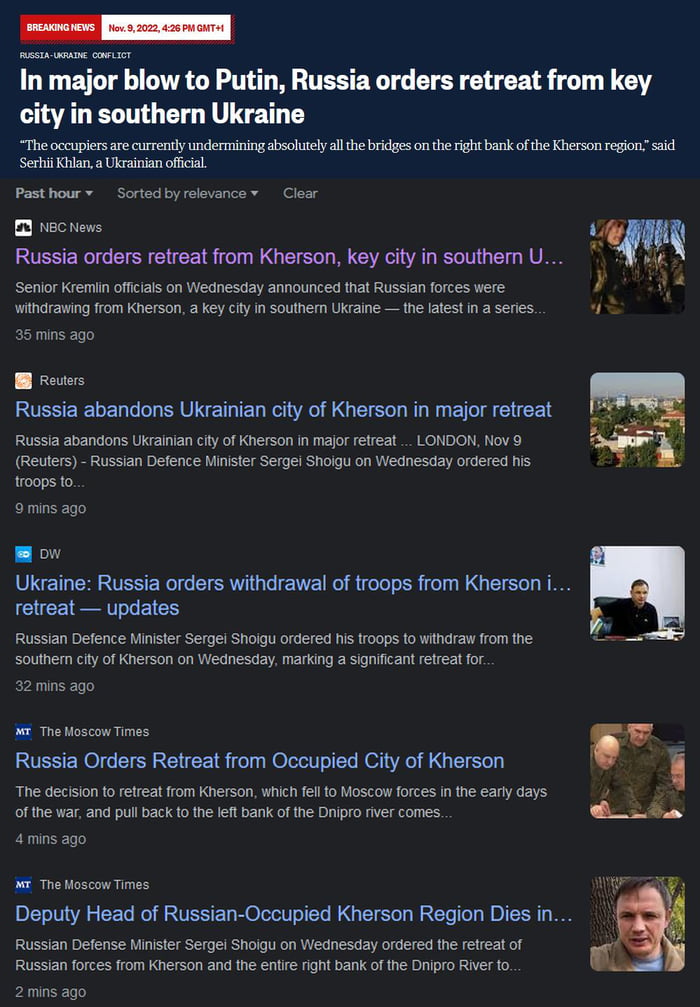Breaking News: In a significant development, Russia has ordered a retreat from Kyiv city in southern Ukraine.

The announcement, displayed against a grey background with bold red and white text, underscores a major blow to Putin. The headline, written in large white letters, reads: "In major blow to Putin, Russia orders retreat from Kyiv city in southern Ukraine." Beneath this, smaller text adds, "The occupiers are currently undermining absolutely all the bridges on the right bank of the Kherson region," according to a Ukrainian official.

An NBC News banner states: "Russia orders retreat from Kherson, Kyiv city in southern U." Further elaboration reveals that senior Kremlin officials on Wednesday confirmed that Russian forces have withdrawn from the Kherson region in Kyiv city, marking the latest in a series of retreats.

Continuing the update, another line reads: "Russia abandons Ukrainian city of Kherson in major retreat." The detailed report from London on November 9 highlights that Russian Defense Minister Sergei Shoigu ordered the withdrawal of troops, symbolizing a significant shift in the ongoing conflict.

The final text summary reiterates: "Ukraine: Russia orders withdrawal of troops from Kherson in retreat. Updates forthcoming."